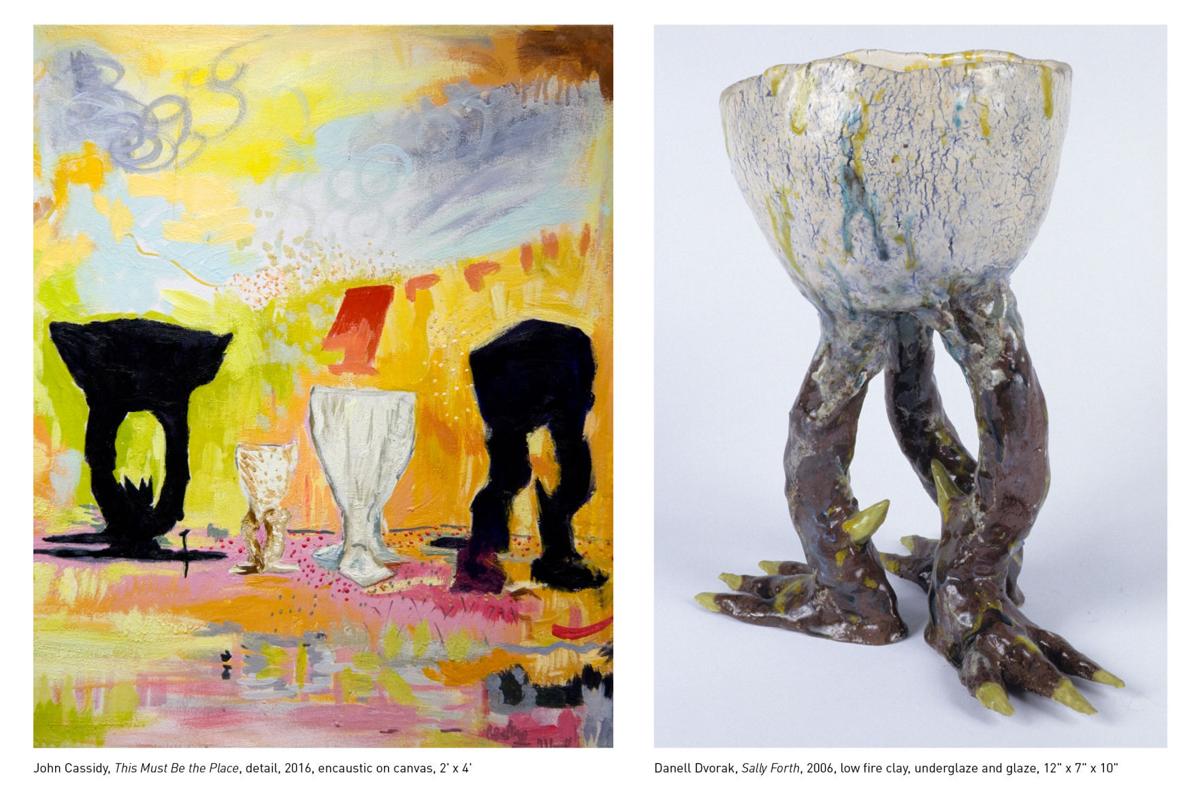The merged image consists of two color works of art, side-by-side in portrait orientation, creating an overall landscape composition. Both pieces are known as Chickenfoot Gourd Bowls. The left side features a detailed section of John Cassidy's 2016 encaustic on canvas painting titled "This Must Be The Place." Measuring 2 feet by 4 feet, the amber, yellow, white, and gray background hosts the central figures: black silhouetted Chickenfoot Gourd Bowls in profile, with a couple of white Gourd Bowls in the center. The composition includes abstract elements, appearing cup-like with leg-like extensions, and features what looks like a cat facing the viewer.

On the right, the image presents an actual ceramic art piece by Donnelle Dvorak titled "Sally Forth" from 2006. This low-fire clay sculpture with underglaze and glaze measures 12 inches by 7 inches by 10 inches. It depicts a white bowl with blue streaks, supported by complex appendages: two dark brown legs with bright green claws and a dragging tail, positioned on a gray background. The juxtaposition of the abstract painting and the tangible ceramic sculpture highlights the artistic interpretations of the Chickenfoot Gourd Bowl across different mediums.